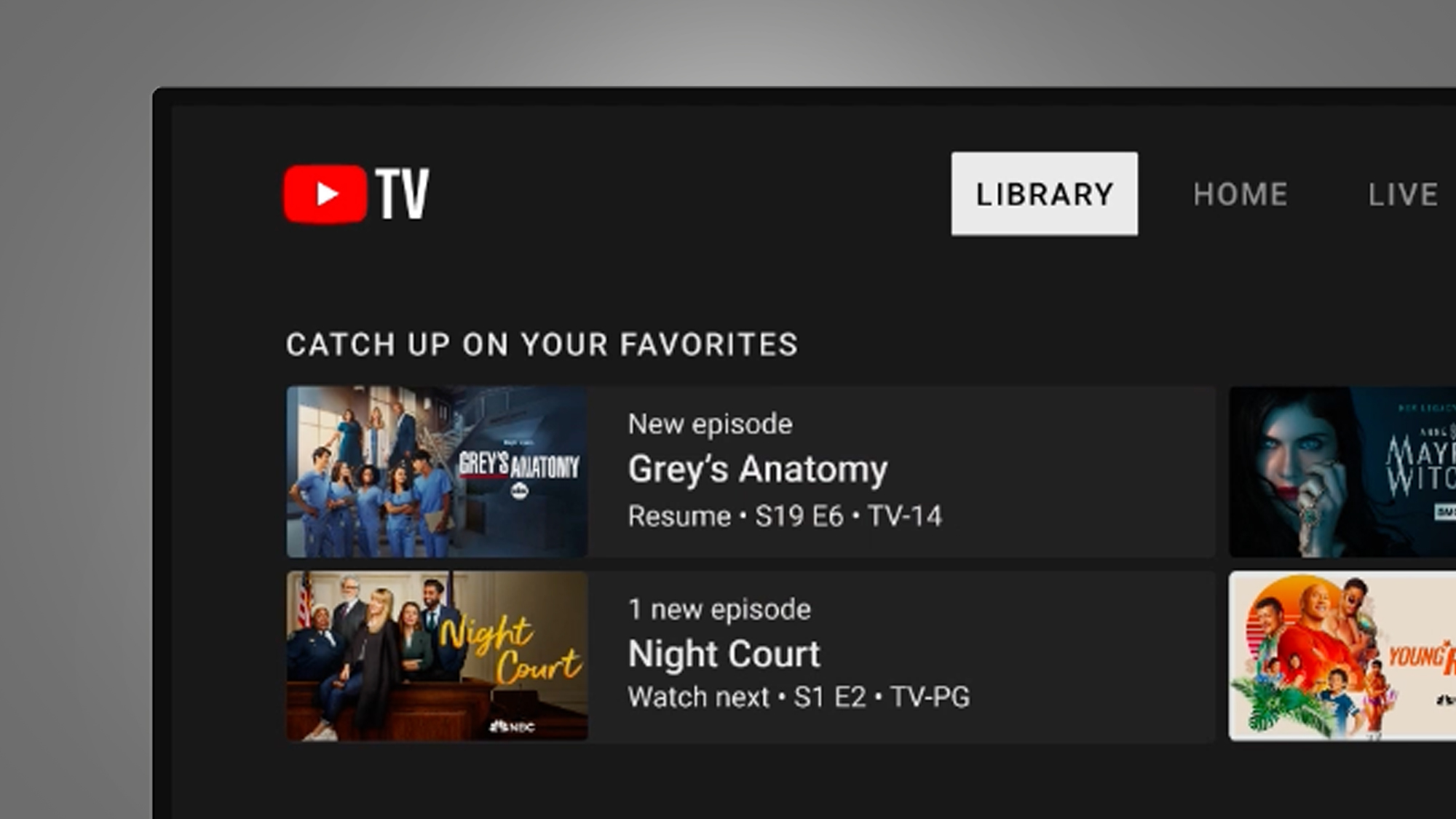This image is a screenshot from a streaming platform, characterized by its dark, black background. In the upper left corner, there’s a red rectangle logo featuring a white triangle pointing to the right. Beside the logo are the letters "TV" in white. The screen is partially cut off on the right and bottom sides, but visible elements offer a glimpse into the platform's user interface.

On the left side of the interface, the highlighted section is labeled "Library" with the subheading "Catch up on your favorites" displayed below it. 

1. The first highlighted show is **Grey's Anatomy**:
    - Network: ABC
    - Season: 19
    - Episode: 6
    - Rating: TV-14
    - Note: A new episode is available.
    - Visual: A still from the show is displayed.

2. The second highlighted show is **Night Court**:
    - Season: 1
    - Episode: 2
    - Rating: TV-PG
    - Note: One new episode is available.
    - Visual: A still from the show is displayed.

To the right of these shows, two more shows or movies are partially visible:
3. One seems to be titled **May Witch**, featuring:
    - Visual: A creepy-looking woman with bluish skin, dark hair, and light blue eyes gazing downwards and holding jewelry.

4. Another show, possibly titled **Young Rock**:
    - Visual: A marketing image on a white background with palm leaves. In the center, a large man wearing an orange or red shirt is surrounded by several other figures:
        - Two men looking over his shoulders.
        - Four younger boys positioned around him.
        - The overall arrangement and aesthetic give off a vibrant, energetic vibe.

This detailed description encapsulates the visual elements and key details from the screenshot, providing a clear understanding of the streaming platform's interface and available content.